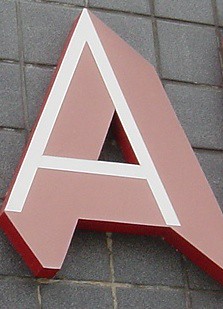The image is a detailed close-up of a tiled surface, likely a floor, though it could feasibly be any flat, square-tiled surface. The tiles are dark grey with a speckled pattern of small white dots uniformly scattered across them. Between each tile are thin cracks filled with a grout material, emphasizing the individual squares and their alignment.

At the center of the image is a three-dimensional letter "A." The design consists of a smaller white "A" layered above a larger "A" that has a light red, almost pink, hue with its sides highlighted in a darker red. This larger "A" creates a shadow effect, giving the illusion that the white "A" is three-dimensional and rising from the underlying surface. The placement of the central triangle in both the white and larger "A" aligns perfectly, enhancing this 3D effect. The contrast between the vivid red border and the solid colors of the letter makes the "A" stand out prominently against the dark, dotted tiles.